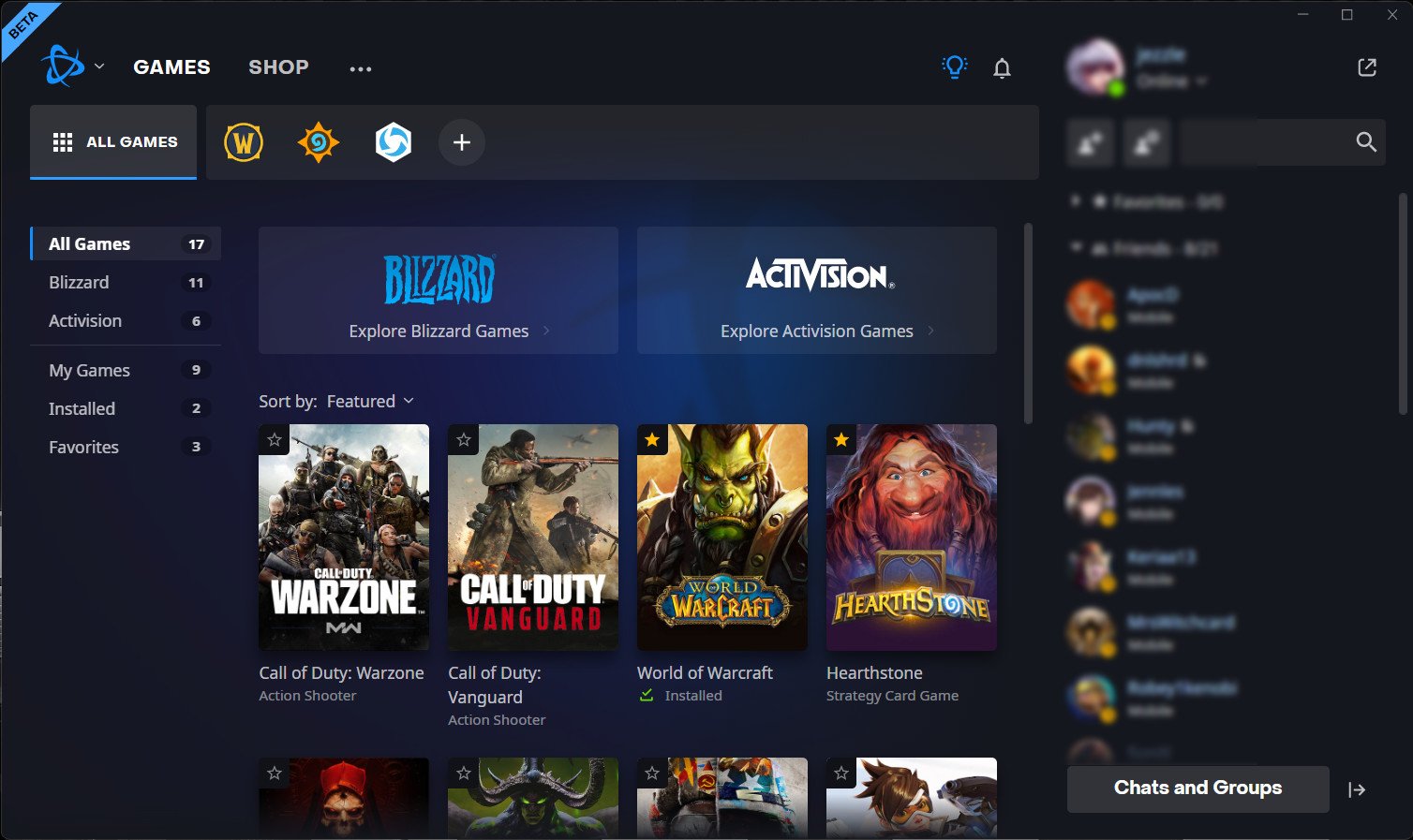The image depicts a website interface with a prominent "Games" header located at the top left corner. The central area features two distinct sections for Blizzard and Activision games on a dark blue background.

On the left side under the Blizzard section, the "Blizzard" logo is styled in blue capital letters with a jagged, icy appearance. Below the logo, the text "Explore Blizzard Games" is written in smaller white letters. This section showcases two smaller pictures:

1. A group of approximately ten soldiers, with the text "Call of Duty" in small white letters above them, and "Warzone" in large, bold capital letters underneath.
2. Two soldiers, one pointing a rifle to the right, with the text "Call of Duty" prominently in large white letters. The word "of" is smaller and positioned between "Call" and "Duty." Below this text is the title "Vanguard" in red letters.

To the right, under the Activision section, the "Activision" logo features an extended "V" that spans over the "C," "T," "I," and "I" in "Activision." Below the logo, there are two more pictures:

1. A green monster with pointy ears staring directly at the viewer, and in front of him is an emblem that reads "World of Warcraft."
2. A man with long red hair, a prominent nose, and a red beard, with an emblem in front of him labeled "Hearthstone."

There is an area to the left of the Blizzard section and to the right of the Activision section showing a blurred section with selections or potential online player images that are not clearly visible. At the very bottom of the image, there are four partially visible pictures, suggesting additional choices.

This website seems to represent a hub for exploring various Blizzard and Activision games.